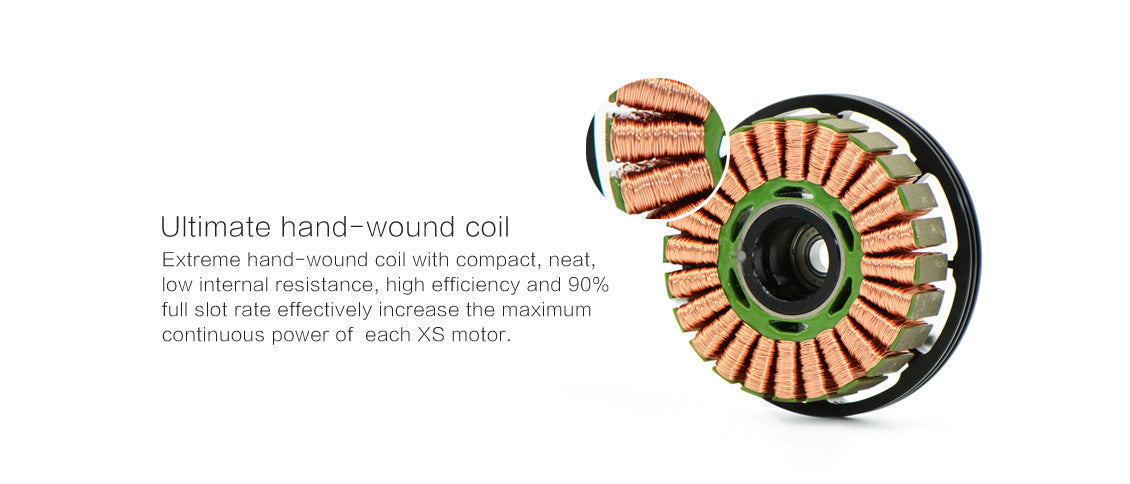The full-color, horizontally rectangular photograph features a hand-wound coil set against a solid white background. Dominating the left side of the image is a block of black text reading "Ultimate Hand-Wound Coil," followed by a descriptive paragraph in a smaller font: "Extreme hand-wound coil with compact, neat, low internal resistance, high efficiency, and 90% full slot rate effectively increase the maximum continuous power of each XS motor." The capitalized "XS" denotes the motor type. Center towards the top is a close-up of three copper coils wound around rectangular shapes, displaying meticulous craftsmanship. On the right side of the image is a larger version of the coil. This coil, composed of numerous copper wires wound in a circular formation resembling a wheel, is anchored by a black metal piece at the back. The coil's assembly includes a green circular core with six symmetrical cutouts—top, bottom, and diagonally. The black band encircling the structure adds a stark contrast, enhancing the intricacy of the copper wiring and the overall compact design.